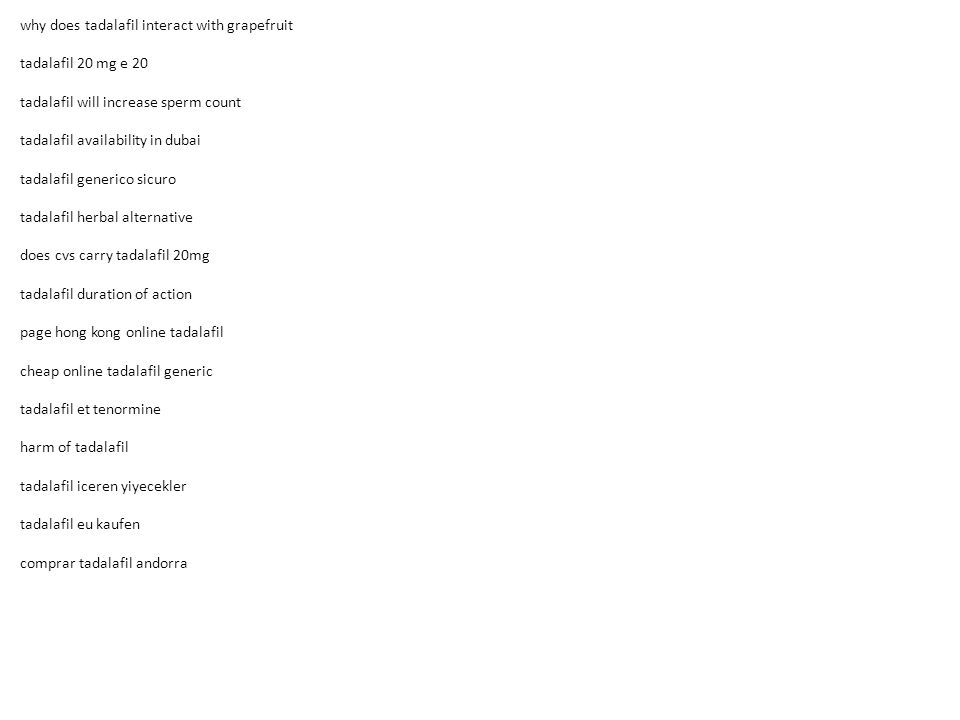**Detailed Caption:**

The image features Tadalafil, a medication commonly used to treat erectile dysfunction, displayed against a clean white background. It highlights various aspects of Tadalafil, including its interaction with grapefruit, which can affect the medication's efficacy. Tadalafil is often available in a 20 mg dosage and has been noted to potentially increase sperm count.

The caption addresses the availability of generic Tadalafil as a safe and accessible option. There are herbal alternatives to Tadalafil for those who prefer natural treatments. Major pharmacies such as CVS carry Tadalafil in the 20 mg strength. 

Additionally, the caption touches upon the duration of action for Tadalafil, making note of its long-lasting effects. For those in specific regions like Hong Kong, there are online platforms where cheap generic Tadalafil can be purchased.

The text provides insights into potential harms associated with Tadalafil usage and lists various names and alternatives linked to the medication, including possibly confusing terms like "iserin," "yeyecler," "eucaffin," "campra," and "indora."

Lastly, a polite "Thank you" concludes the detailed and informative caption.